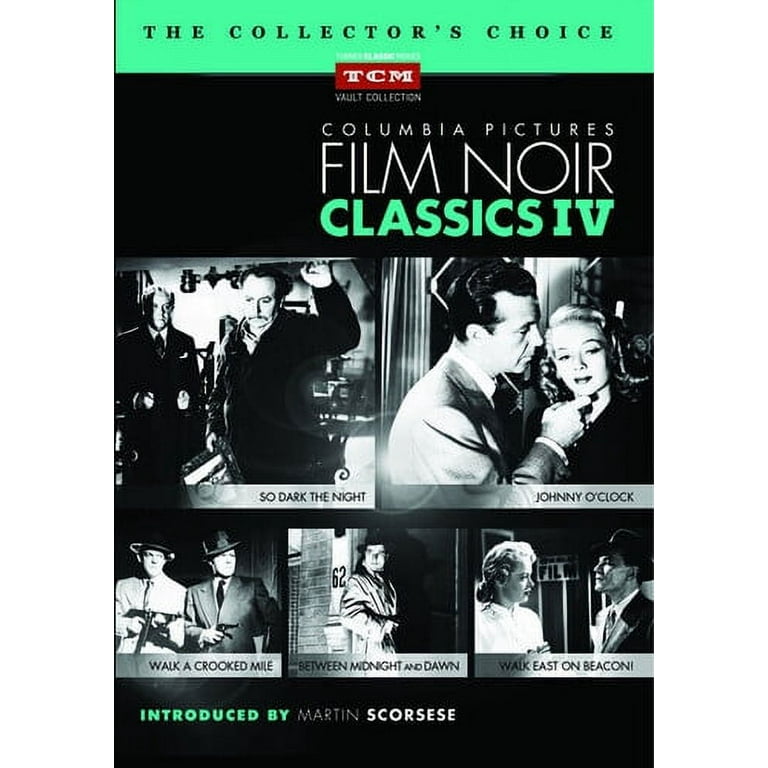This image is a promotional poster from the TCM Vault Collection, showcasing the "Columbia Pictures Film Noir Classics 4," a collector's edition DVD set presented by Turner Classic Movies (TCM). The poster features a black background with the text "The Collector's Choice" highlighted in light green, along with black-and-white tones dominating the overall design. At the top, it proudly displays "Columbia Pictures Film Noir Classics 4" in large font, and at the bottom, it mentions that the collection is introduced by famed director Martin Scorsese. The set includes five iconic film noir movies: "So Dark the Night," "Johnny O'Clock," "Walk a Crooked Mile," "Between Midnight and Dawn," and "Walk East on Beacon." This edition is a must-have for collectors and enthusiasts of classic film noirs.